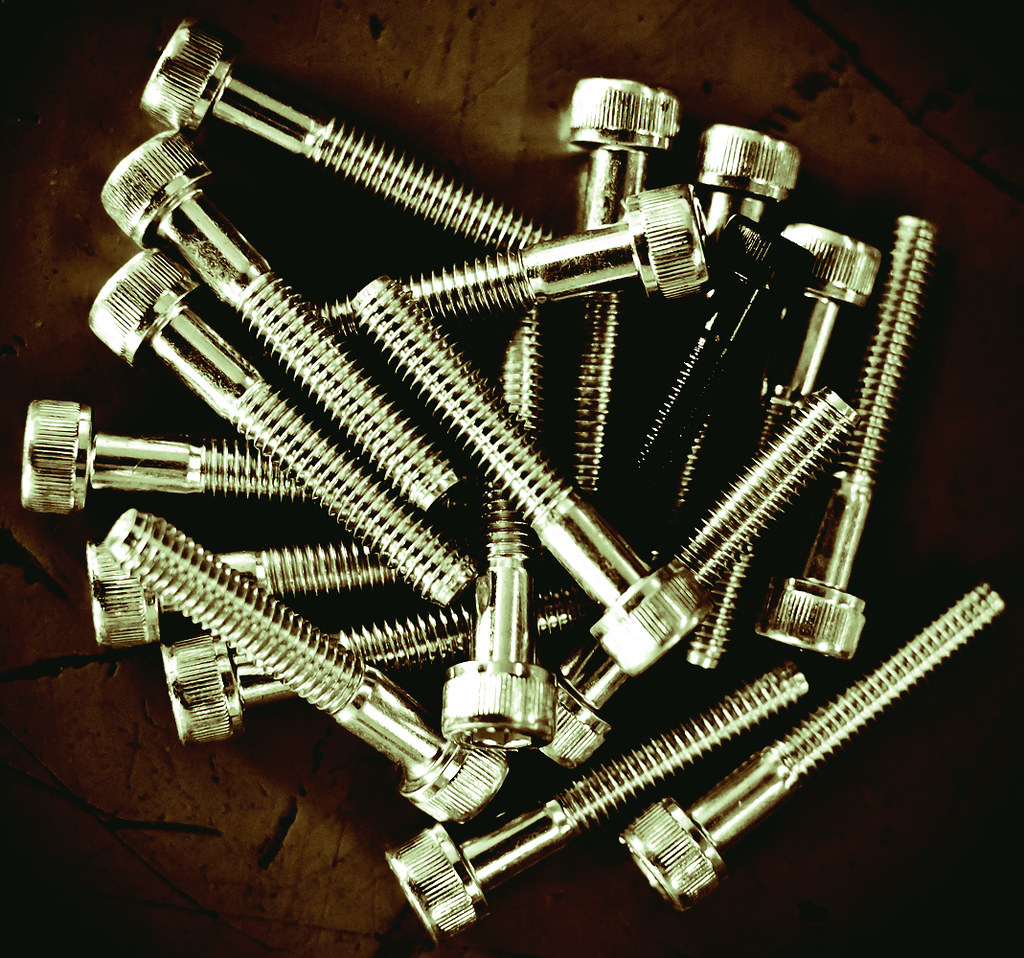In the image, a pile of screws, possibly bolts, lies jumbled together on a slightly ambiguous dark brown background that might be a wooden tabletop. The screws are primarily silver, though there is one black bolt nestled towards the center of the image, creating a stark contrast. Each screw features a knob at the top followed by a smooth portion and then finely machined threads that run at least three-quarters of their approximately two-inch length. The lighting, coming from the left side, casts shadows to the right, enhancing the metallic texture and giving some screws a gold-like hue. Reflections play across the shiny surface, especially highlighting the top of a central silver screw. The photograph maintains clear focus throughout, ensuring all details are crisply captured.